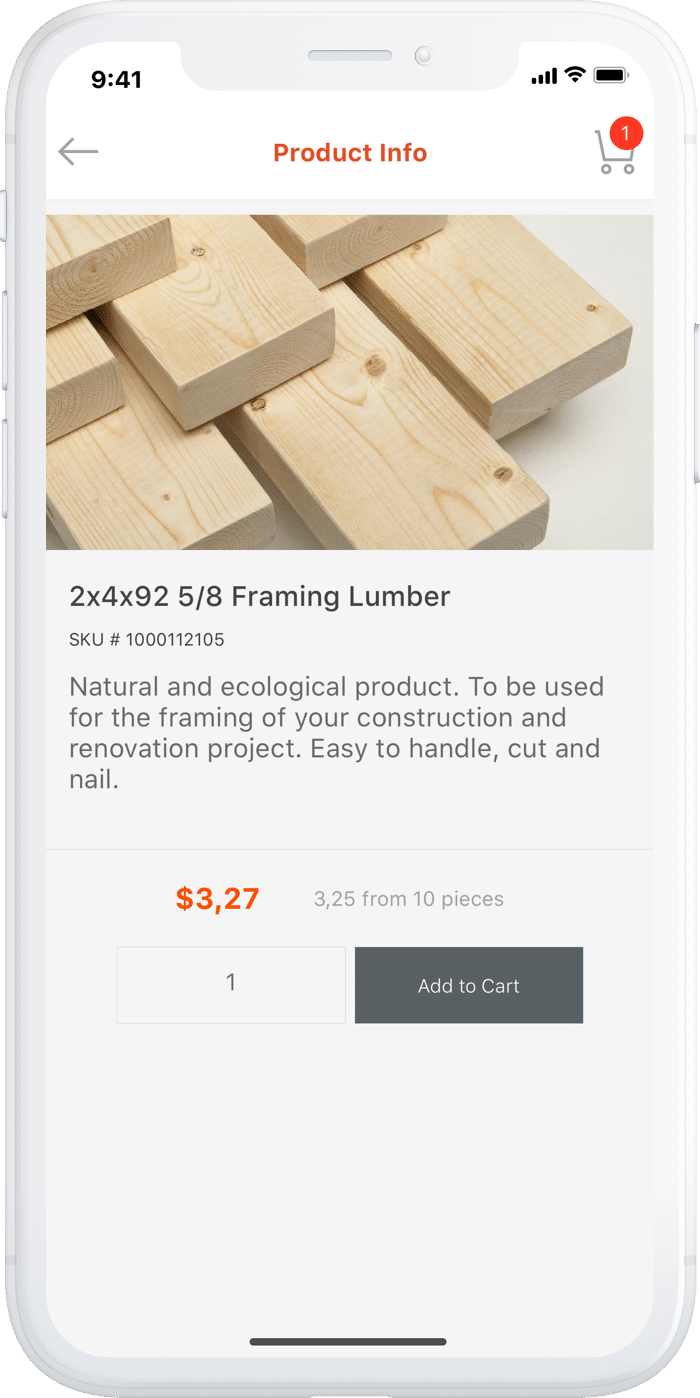**Detailed Product Page Description:**

The image is a screenshot of a product page showcasing a specific type of construction material. At the top of the page, a heading in orange text reads "Product Info." Adjacent to this text on the right side, there is a cart icon with an orange circle indicating that there is one item in the cart, marked with a white number "1" inside the circle. On the left side of this section, a grey back arrow icon allows users to navigate to the previous page.

Below this header section, there is a picture of wooden 2x4s, providing a visual representation of the product available for purchase. Underneath the image, the product is labeled as "2x4x9 2 5/8' Framing Lumber," followed by the SKU number: 1000112105. The product description emphasizes that it is a natural and ecological option, suitable for framing in construction and renovation projects. It highlights that the lumber is easy to handle, cut, and nail.

The price of the lumber is prominently displayed below the description, listed as $3.27 per unit. Directly beneath the price, there is a button labeled "Add to Cart." To the left of this button, there is a quantity field set to the default number "1," allowing users to specify the number of units they wish to purchase. The entire section is set against a clean, white background.